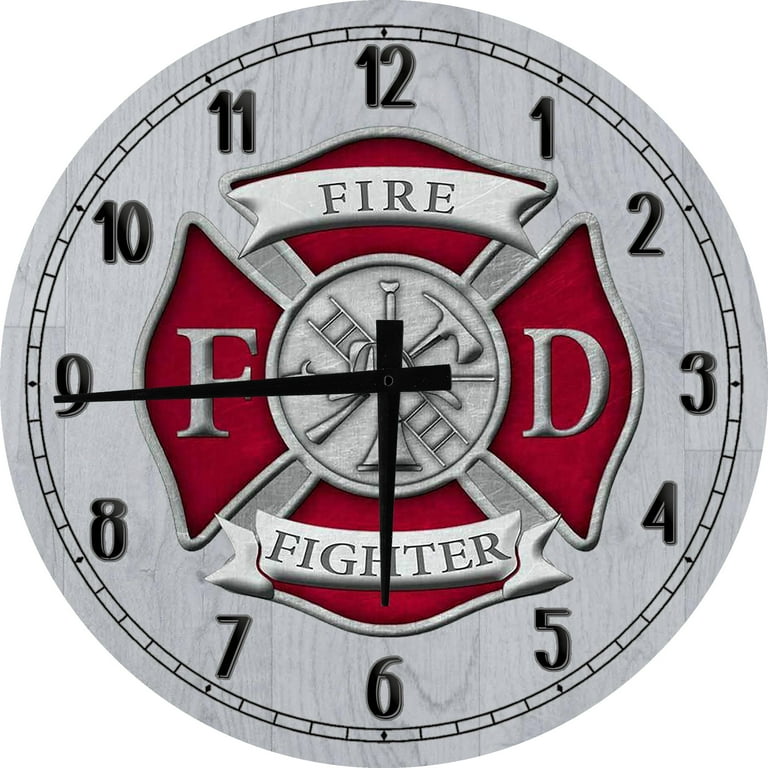The image features an analog wall clock with a gray wooden background that mimics the texture and markings of a typical wooden floor. The face of the clock displays black numbers from 1 to 12, with black minute and hour hands currently pointing to 6:45. 

Central to the clock’s design is a red four-pointed emblem with a silver outline, resembling a cross. This emblem is emblazoned with the firefighter insignia - tools commonly used in firefighting, including a ladder, a hatchet, and potentially a hose nozzle and pike, all crossed to form an X. The emblem also contains a silver circle at its center. 

On the left and right points of the red cross are the letters F and D, representing the fire department, rendered in silver. The top and bottom points feature silver banners with the words "Fire" and "Fighter" respectively, in darker black lettering. The clock hands obscure part of this central image, adding depth to the intricate design. The clock’s rim appears either painted with or embossed to give a highlighted effect around the logo.